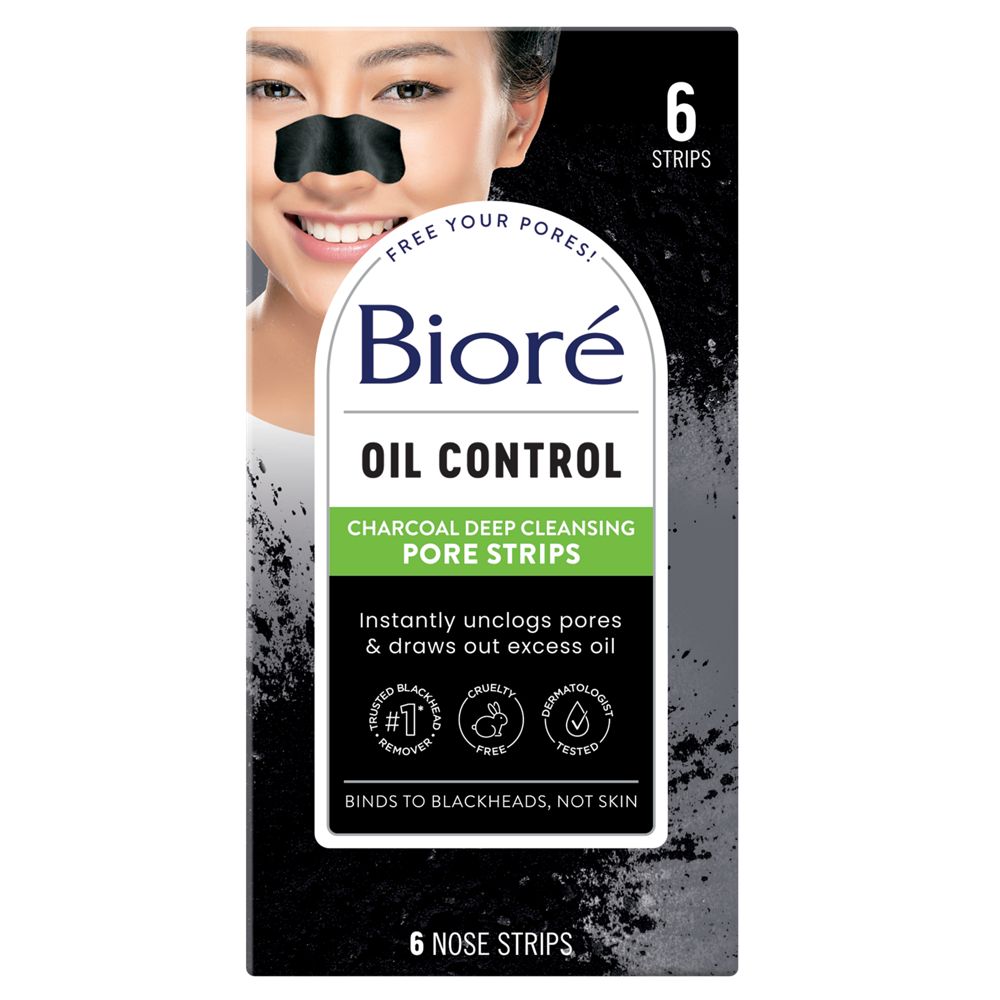The image is a tall, narrow advertisement for Biore Oil Control Charcoal Deep Cleansing Pore Strips. Dominating the upper left corner is a model, a Caucasian female with dark brown, pulled-back hair, wearing a white top. She is pictured facing the viewer with a black pore strip horizontally across the bridge of her nose. The packaging features a prominent label that includes the following key details: "Biore oil control charcoal deep cleaning pore strips," and in a black background with white text, it reads, "instantly unclogs pores and draws out excess oil." 

There are several badges and claims across the image indicating the product is "cruelty-free," "dermatologist tested," and a "number one remover." The packaging also emphasizes that the strips "bind to blackheads, not skin," and the product includes "six nose strips" noted both at the bottom and in the upper right corner in white text. The visual design has sections with white, black, and hints of green, particularly noticeable around the detailed descriptions and logo, giving it a clean yet striking appearance. The overall theme focuses on the efficacy and essential benefits of using the charcoal-based pore strips.